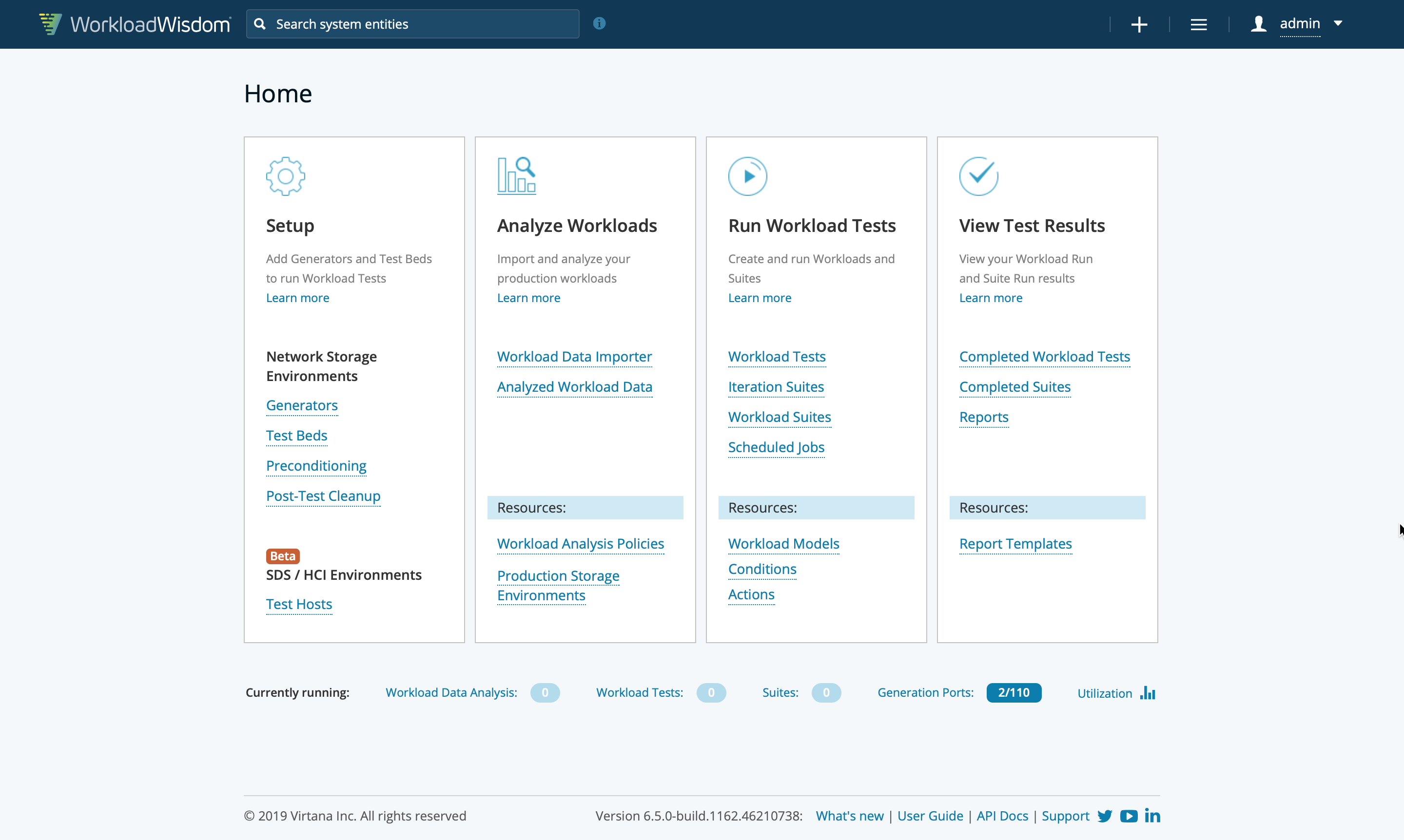**Caption**: "This image displays the detailed interface of the Workload Wisdom Dashboard. At the top, the interface features a search bar labeled 'Search System Entities.' Below that, a navigation menu provides various options starting with:

- 'Home'
- 'Set up your Administrator Account'
- 'Set up Home Network'
- 'Home Network Storage Environments'
- 'SDS ACI Environments'

Further down, the menu includes options to:

- 'Analyze Workloads'
- 'Resources'
- 'Workload Data'
- 'Prompter Importer'
- 'Analyze Workload Data'

Continuing, it lists resources for:

- 'Workload Analyst Policies'
- 'Production Storage Environments'

The dashboard also includes functions to:

- 'Run Workload Tests'
- 'Schedule Jobs'
- 'Workload Models'
- 'Conditions and Actions'

Lastly, the interface provides options to:

- 'View Test Results'
- 'Completed Workload Tests'
- 'Completed Suites'
- 'Reports and Resources'
- 'Report Templates'

This dashboard clearly serves as a comprehensive tool for administrating and analyzing workloads, likely designed for IT professionals managing complex network and storage environments."